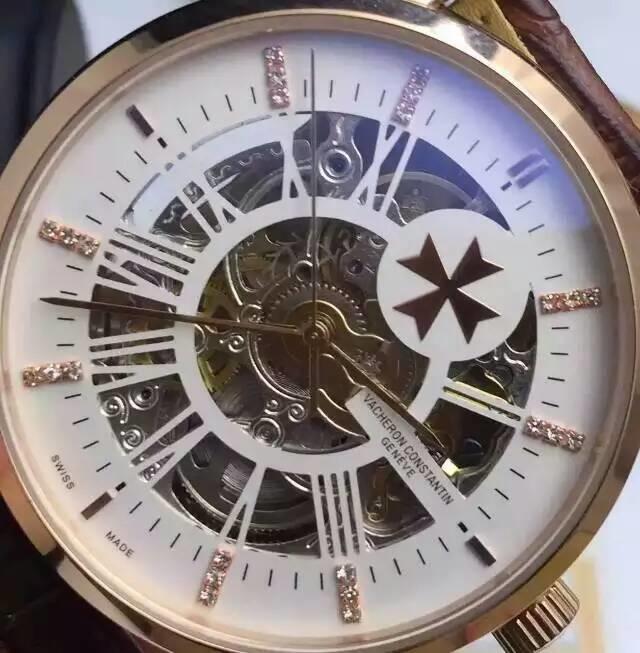The image features a detailed close-up of the face of a luxurious wristwatch. The watch has a gold-toned outer ring and a winding knob on the right side. It is adorned with a brown leather strap that is partially visible at the top edge of the image. The watch’s face is white with a clear, small opening in the middle, revealing the intricate, silver gears and inner workings of the timepiece. 

The hour markers consist of sparkling, diamond-like rectangular lines, and these gleaming markers are positioned at the 12, 1, 4, 5, 7, 8, 9, and 10 o'clock positions. The 2 o'clock position features two black strips, while the remaining hour markers are marked with single black strips. The silver minute and hour hands point to approximately 3:43, with the second hand slightly past the 11th hour mark. 

The watch prominently displays the brand name "Vacheron Constantin" along with "Geneve" in text on the face. Additionally, there is a distinctive cross-like symbol with thicker outer edges within a white circle on the right side. Overall, the image captures the elegance and precision-engineering of this exquisite timepiece.